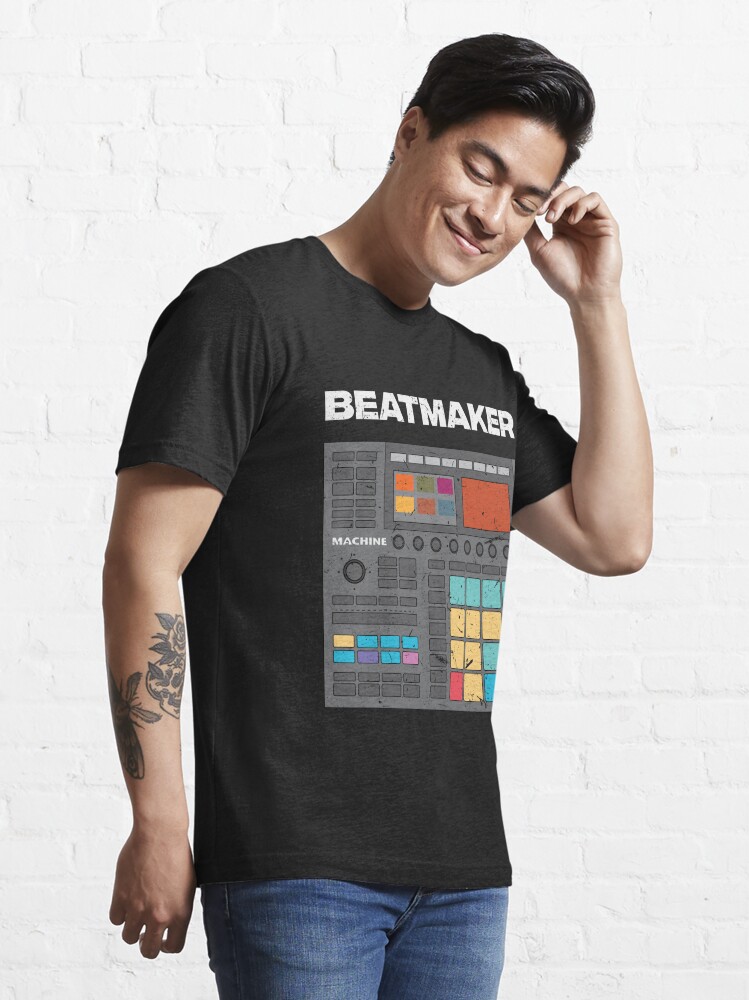A photo of a man taken indoors against a white brick wall. The man, who appears to be in his late 20s and possibly of Asian descent, stands at the center of the image with a slightly tilted head and a satisfied smile. His eyes are closed. He has dark brown hair and is dressed in a black short-sleeved t-shirt and blue jeans. The black shirt features the word "Beatmaker" in white font above an illustration of a DJ apparatus or electronic turntable, complete with various colored buttons and switches, predominantly in yellow and blue. His left hand is touching his ear while his right arm displays tattoos, including a floral design. He exudes a confident and artistic vibe, likely indicative of his occupation as a DJ or music artist.